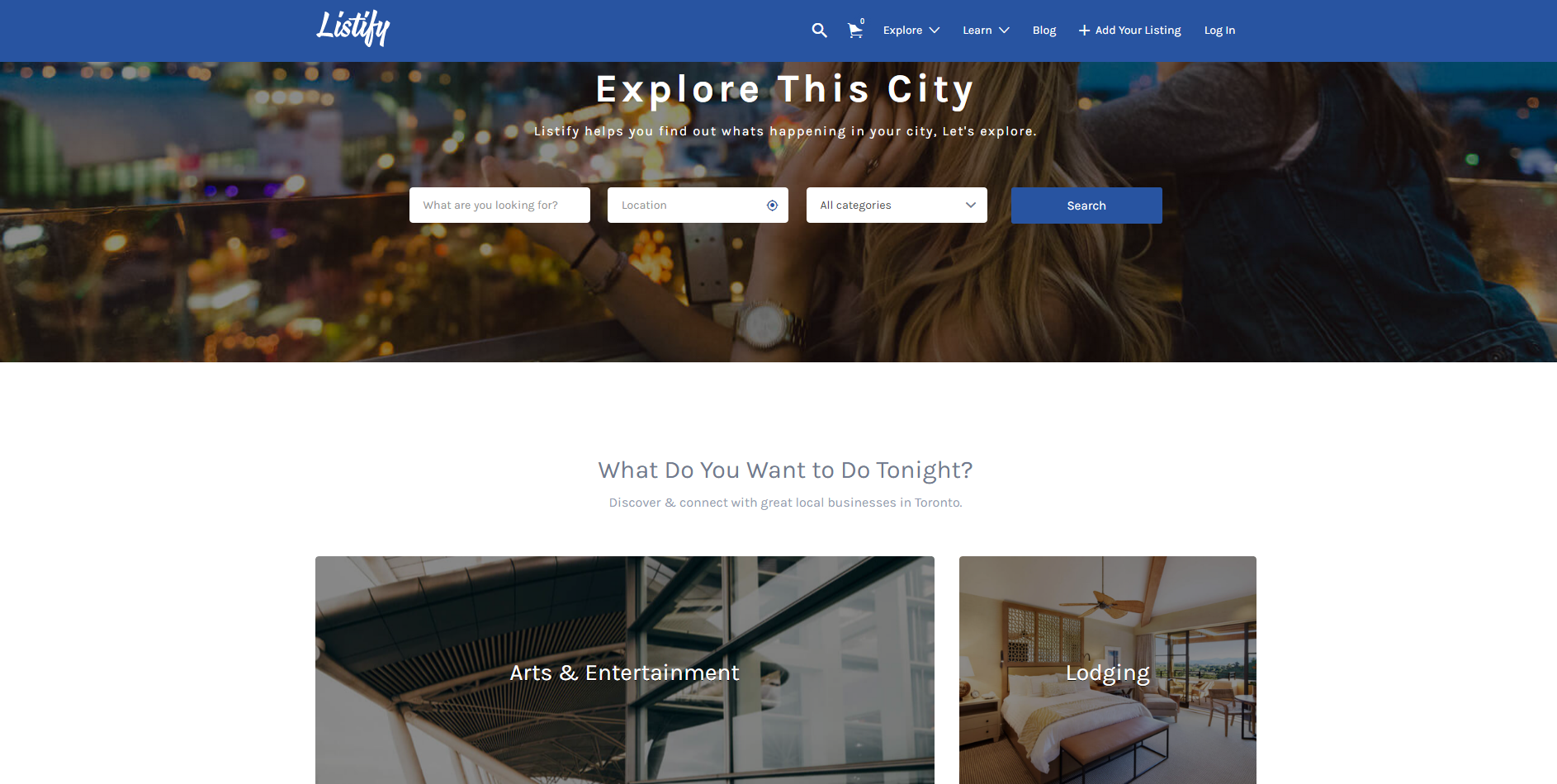A screenshot from Listify, an online platform for discovering local events and businesses, showcases its homepage interface. At the top, a dark blue header prominently features a magnifying glass, a shopping cart icon, and navigation options labeled Explore, Learn, Blog, Add Your Listing, and Login. Below the header, a large rectangular cityscape image captures two individuals gazing upward from an elevated vantage point, accompanied by the motivational text: "Explore this city. Listify helps you find out what's happening in your city. Let's explore."

Beneath the cityscape banner, a search interface is presented with text boxes for "What are you looking for?" and "Location," along with a dropdown menu labeled "All Categories" and a blue search button. Further down the page, a section titled "What do you want to do tonight?" invites users to discover and connect with noteworthy local businesses in Toronto.

This section features two visuals: a wide rectangular image labeled "Arts and Entertainment," depicting the interior of an unspecified building, and a square image labeled "Lodging," showcasing a hotel room with a focus on a neatly made bed. The design and content collectively aim to engage users in exploring and connecting with their city's dynamic offerings.